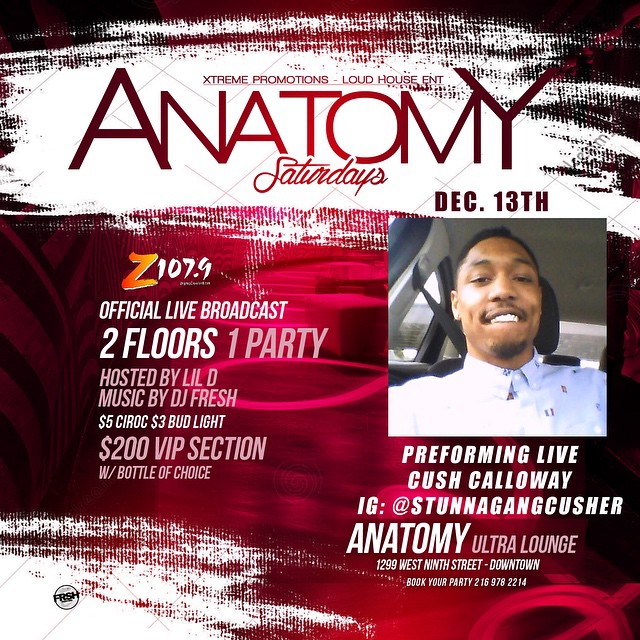This promo poster for an event features a striking design with a scratched red background and a white section for the text. The header reads "Extreme Promotions, Loud House Entertainment, Anatomy Saturdays," followed by the date "December 13th." To the right, there’s a photo of an African American gentleman, possibly in his early 30s, smiling in the passenger seat of a car and wearing a white button-up shirt with red and blue embroidery. The text "Performing Live, Cush Callaway" appears next to him, along with his Instagram handle "@StunnaGangCusher." The event will be hosted at Anatomy Ultra Lounge, located at 1299 West 9th Street, Downtown. Additionally, the poster notes an official live broadcast by Z107.9, featuring Lil D as the host and music by DJ Fresh. Attendees can enjoy $5 Ciroc and $3 Bud Light. VIP sections are available for $200, which includes a bottle of choice. There's also a contact detail for booking parties, although the text is too small to read clearly.